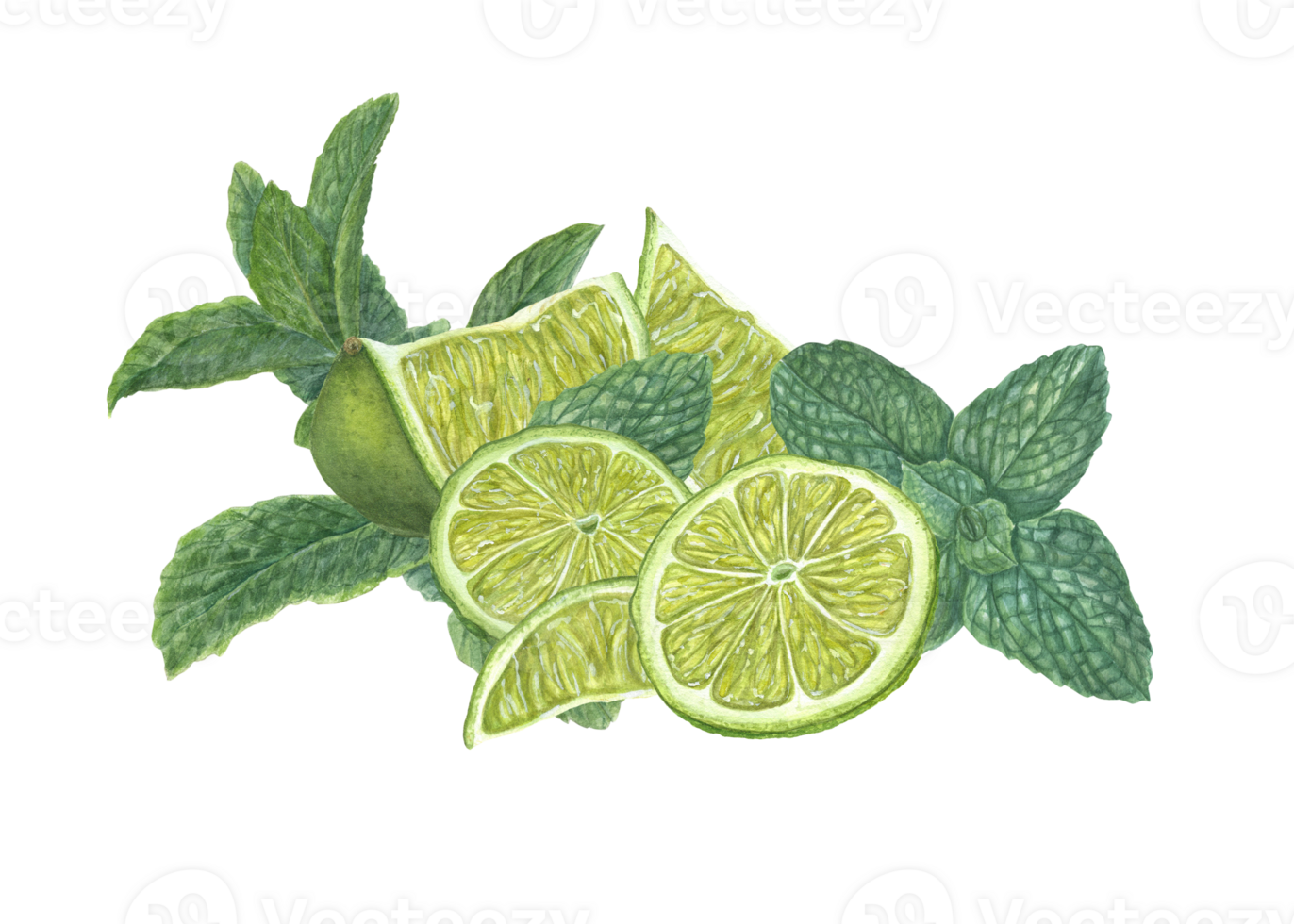This detailed image portrays a vibrant, hand-drawn depiction of cut limes set against a pure white backdrop, which features a subtle watermark with a circular design and the text "Vecteezy." Central to the composition are multiple sections of lime fruit: two thinly sliced circular pieces and several quartered wedges showing the intricate texture of the white pith and the light green-and-white juicy interiors. Surrounding the limes are varying green leaves, including a prominent three-pronged leaf to the right and darker evergreen leaves interspersed among the lime slices. The precise sketching highlights the small details of the citrus pulp, giving the entire artwork a somewhat cartoonish yet realistic feel, reminiscent of something you might see as garnish in a cocktail.